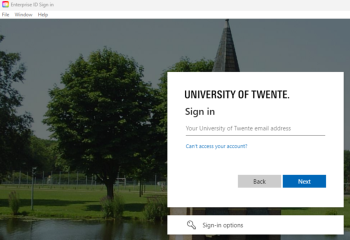Screenshot of a login page on a website with a park-themed background tinted dark for emphasis. A white login window occupies the bottom right corner, prominently featuring the "University of Twente" title. The interface begins with a "Sign in" instruction followed by a text field labeled "Your University of Twente email address." Directly beneath, a blue hyperlink reads "Can't access your account." A gray "Back" button and a blue "Next" button are aligned horizontally below this text field. Following these options, another white rectangular section at the bottom denotes "Sign in options."